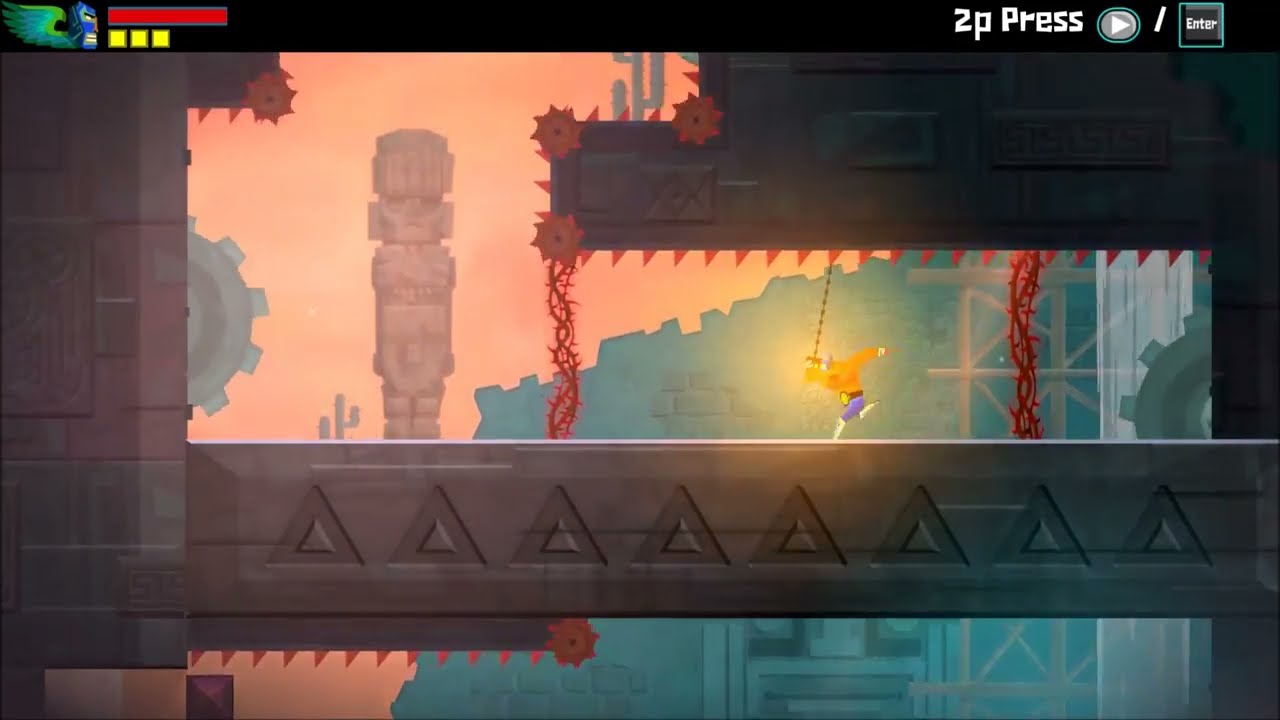The image is a detailed screenshot from a cartoonish 2D video game with a desert-themed background featuring cactuses, mountains, and several mechanical elements such as gears and lights. In the center of the screen, two characters are visible: an orange-toned wrestler wearing blue shorts and a mask, resembling a WWE outfit with a prominent belt buckle, and a flame-engulfed creature with four legs, potentially an animal, located towards the bottom left corner. The top of the screen displays a health bar at the center, which is green and about 25% full, depicted within a bone shape flanked by two skulls. To the left, there is a cartoon eagle icon with a red health bar and three yellow squares underneath, possibly indicating additional player stats. The top right corner of the screen shows control instructions in white text, indicating "2P press" alongside a right arrow and an entry key.